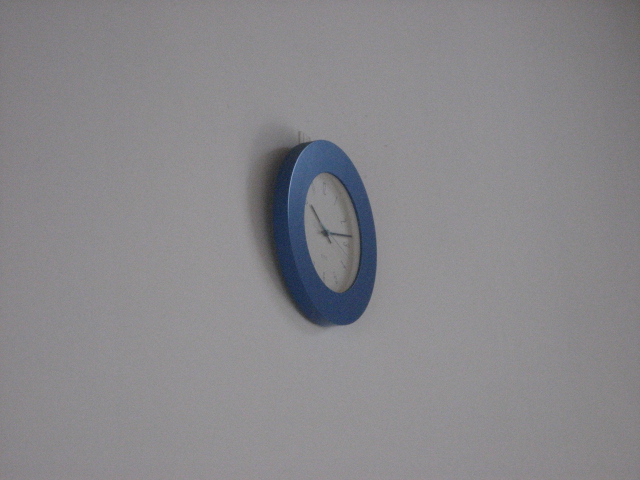A slightly blurry photograph captures a round clock mounted on a stark white wall. The clock features a beveled edge in a striking cobalt blue. Its white face is adorned with traditional Roman numerals, while slim black hands indicate the time as approximately 10:13 or 10:14. The clock is hanging from a visible hook, and the image is taken from an angle, offering a partial side view of the left edge of the clock. There are no other elements present in the composition, emphasizing the clock's simplicity against the plain background.